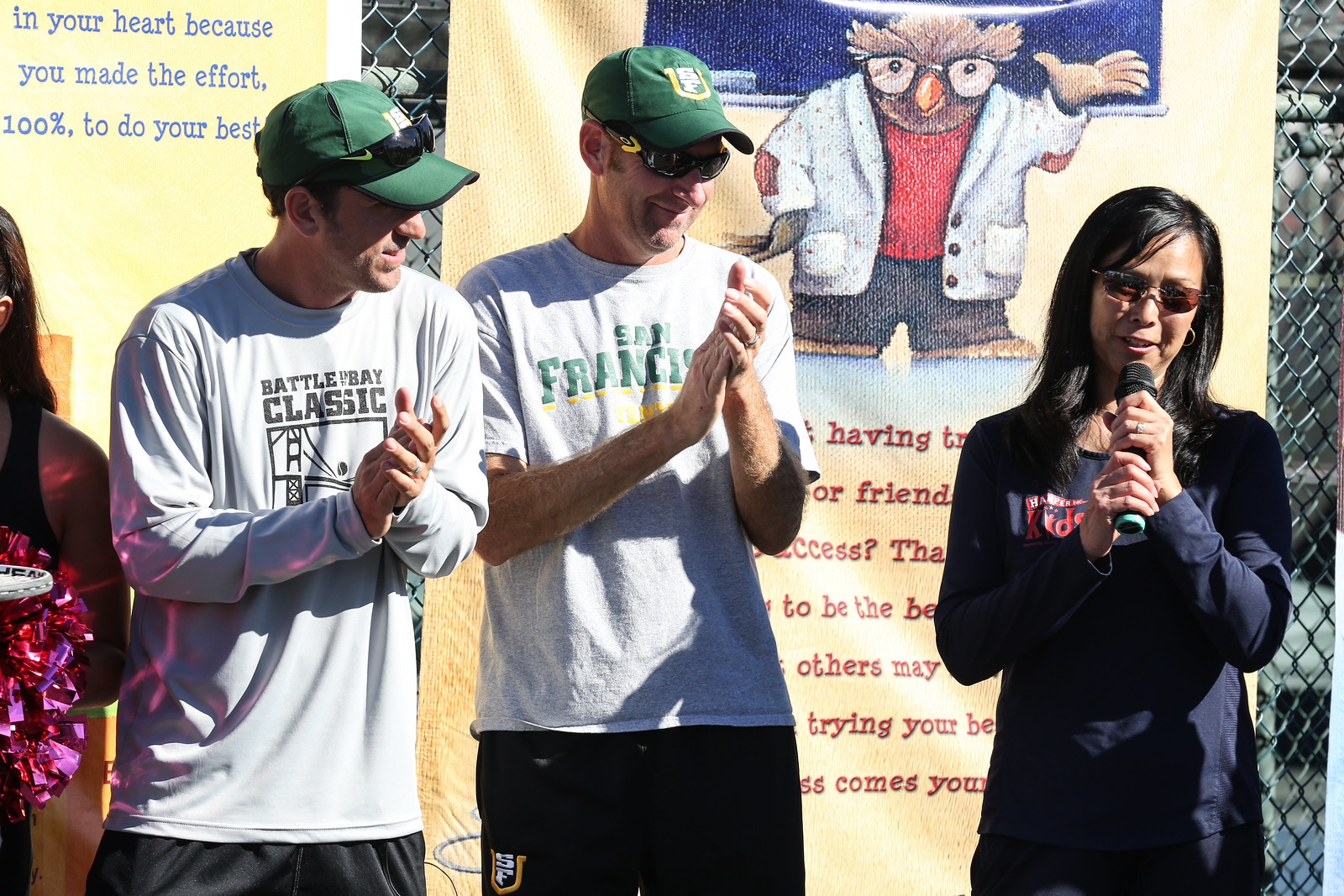This photograph captures an outdoor community event, possibly a children's charity or an awards ceremony. Central to the image are four individuals. In the foreground, a light brown-skinned woman stands on the right, dressed in a dark suit and sunglasses, holding a microphone and seemingly speaking. To her left, two men in gray t-shirts adorned with green and black lettering—one reading "Battle of the Bay Classic" and the other "San Francisco"—and green hats associated with the San Francisco Dons men's basketball team, are clapping with their hands positioned in front of them. Both men have sunglasses, with one wearing them and the other having them perched on his hat. On the far left, partially cut off, another person, possibly female, appears to be holding pom-poms. Behind them, vibrant signage featuring a cartoon owl and various motivational texts, though partially obscured, dangles from a chain link fence, contributing to an upbeat atmosphere. Notable readable phrases on the signs include, "In your heart, because you made the effort 100% to do your best." The collective focus of the group is directed towards the woman with the microphone, enhancing the image's sense of community and inclusivity.